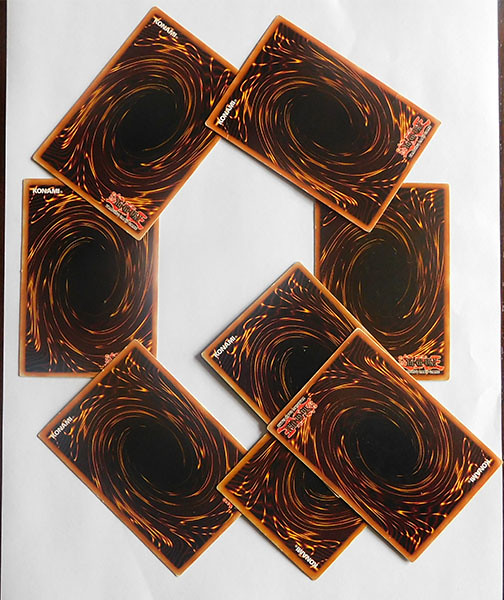In this image, there are eight cards resembling baseball or postcard-sized items, each designed with an intricate tornado-like swirl pattern. The swirl features varying shades of brown and orange, with a defining black center, while the edges of the cards have a light brown border. The cards display some white and red lettering, although the exact text is not clear. These cards are arranged in a circular formation on a bright white backdrop, giving the impression of a product display, potentially for a website. The swirling design evokes the visual of a wave curling down. The overall setup is clean, emphasizing the consistent and striking pattern of the cards against the minimalist background.